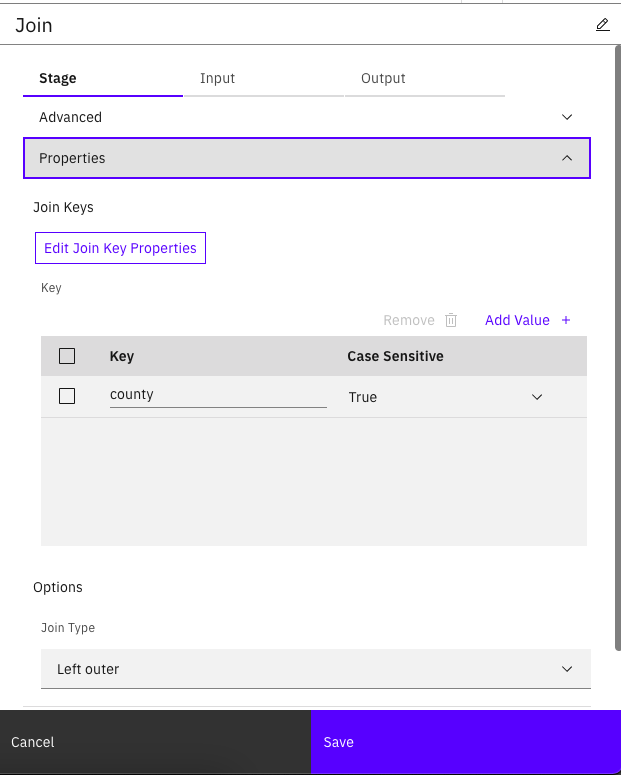This screenshot displays the backend interface of a software or website. At the top, there's a banner with the label "Join." Directly beneath this banner is a line, and below that, within the same section on the far right, there is a pencil icon. Just under this section, there are three tabs labeled "Stage," "Input," and "Output," with the "Stage" tab highlighted in blue. 

Further down, the text "Advanced" appears, accompanied by a dropdown arrow symbol on the far right side. Below this, the section titled "Properties" stands out, highlighted by a blue outline and featuring an upward arrow icon to indicate that it can be collapsed, located on the far right.

At the bottom of the screenshot, there's an area titled "Join Keys," which is enclosed in a blue box. Within this area, the text "Edit Join Key Properties" is displayed in blue, signifying that it is a clickable link or button for further actions.